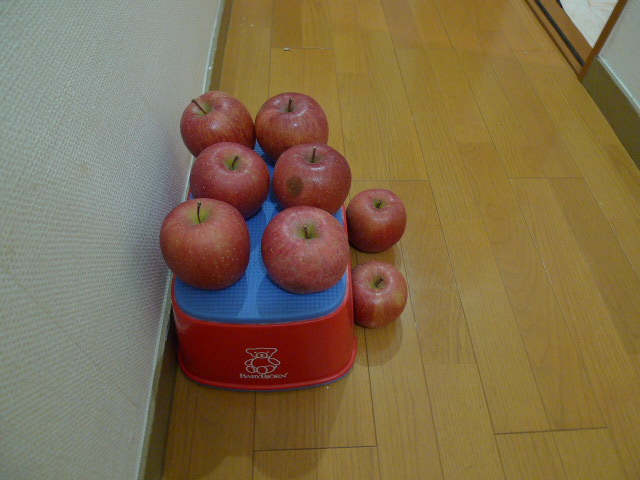This color landscape photograph shows a group of eight red apples with brown stems, prominently displayed in what appears to be a home passageway. Six of the apples are arranged neatly on a blue pad that rests atop a red container featuring a white logo. The other two apples are placed directly on the light brown parquet floor, just below the container.

The scene is bordered by walls that exhibit distinct features, adding depth to the setting. The left wall appears teal green with a subtle pattern, contrasting with the far-right teal wall which has a dark green baseboard at the bottom. Near the container, the flooring and baseboard are clearly visible, providing additional context to the indoor environment. This passageway likely features a textured surface on both walls, contributing to the overall cozy yet slightly eclectic atmosphere. The arrangement of the apples, combined with the intricate details of their surroundings, creates a compelling visual that captures a moment of serene domesticity.